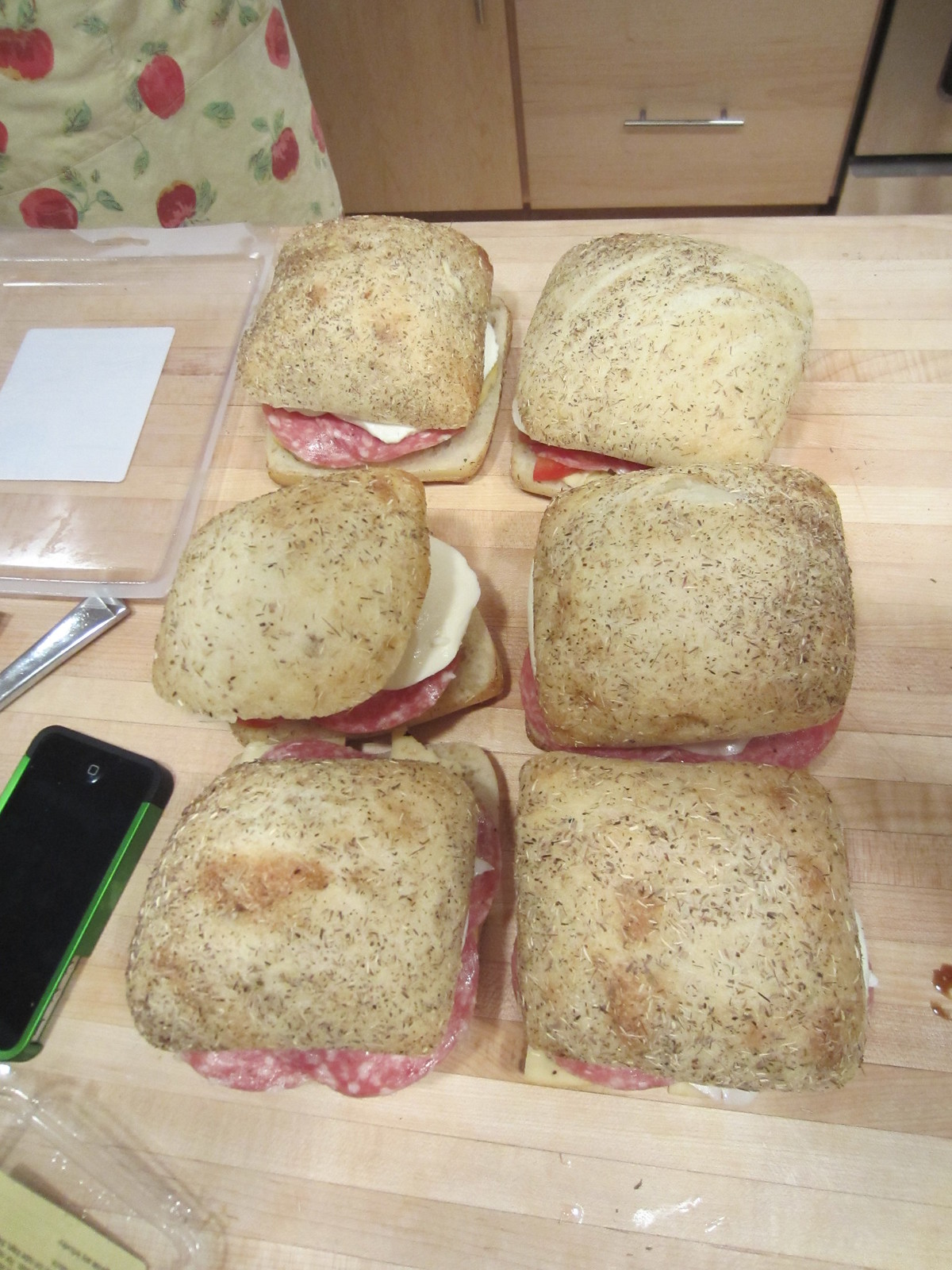This color photograph captures a neatly arranged composition within a kitchen setting. At the center lies a trio of orderly pairs, making a total of six toasted sandwiches featuring white cheese and sliced salami on Shabbat bread, displaying small black seeds typically seen in rye bread. These delectable-looking sandwiches are placed on a light-colored wooden countertop, partially covered by a piece of plastic wrap. Adjacent to the sandwiches on the left side, there's a cellphone enclosed in a green and black case, a transparent plastic lid with a white label facing down, and a piece of silverware, likely a fork or knife. The scene includes visible elements of the kitchen: a lower drawer with a silver handle, light brown cabinets in the background, and a printed kitchen cloth adorned with apple prints positioned on the top left. A possible lady's apron with a white background and large red strawberries with green leaves can also be discerned. The overall atmosphere is one of a cozy and active kitchen moment.